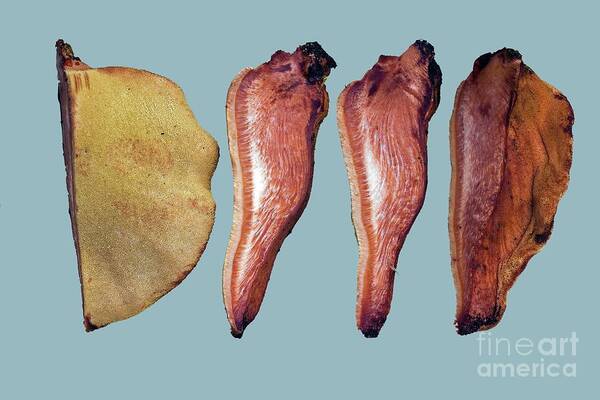This color photograph, set against a light blue background, showcases four distinct objects. In the lower right corner, the text "Fine Art America" appears in lowercase, white lettering. The objects seem to be pieces of leather or anatomical representations in various stages. 

The first object is a semi-circular shape with a textural light brown to yellowish coloring and includes a straight brown line extending from it. The second object, shaped similarly to a tongue, is primarily dark brown with hints of reddish-pink hues. The third object, reminiscent of a small beaver’s face, is dark brown and identical in shape and size to the second object. The final and largest object differs in both shape and coloration, being wider, less uniform, with a darker brown color and a pink streak down the middle. Together, these objects create a visually intriguing and textured composition.